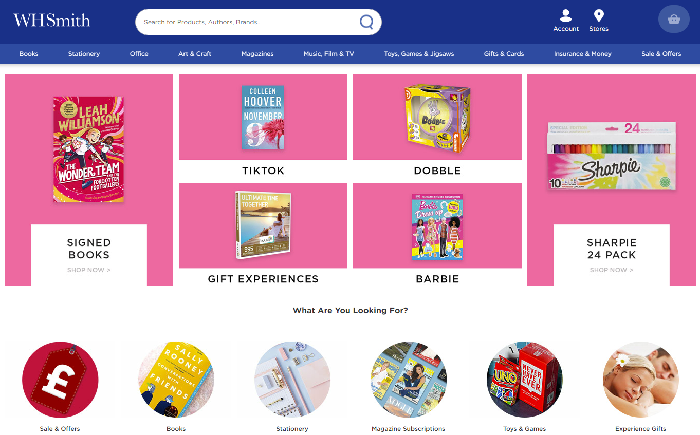The WHSmith website interface is depicted in this image. At the top, within a blue panel, there's a prominent search bar allowing users to enter queries. To the right of this, there are buttons for account access and finding stores, along with a shopping cart icon. Just beneath the WHSmith logo and the search bar, an array of subheadings offers quick navigation to specific sections including Books, Stationery, Office, Art and Craft, Magazines, Music, Films and TV, Toys, Games and Jigsaws, Gifts and Cards, Insurance and Money, and Sales and Offers.

In the central area of the screen, against a backdrop of alternating pink shades, highlighted items are displayed. Featured products include signed books, Barbie dolls, and a 24-pack of Sharpie double-ended pens.

Towards the bottom of the page, there are additional link icons that duplicate the categories found in the top navigation bar, designed to catch the eye and provide convenient access. These include Sales and Offers, Books, Stationery, Magazine Subscriptions, and Toys and Games.